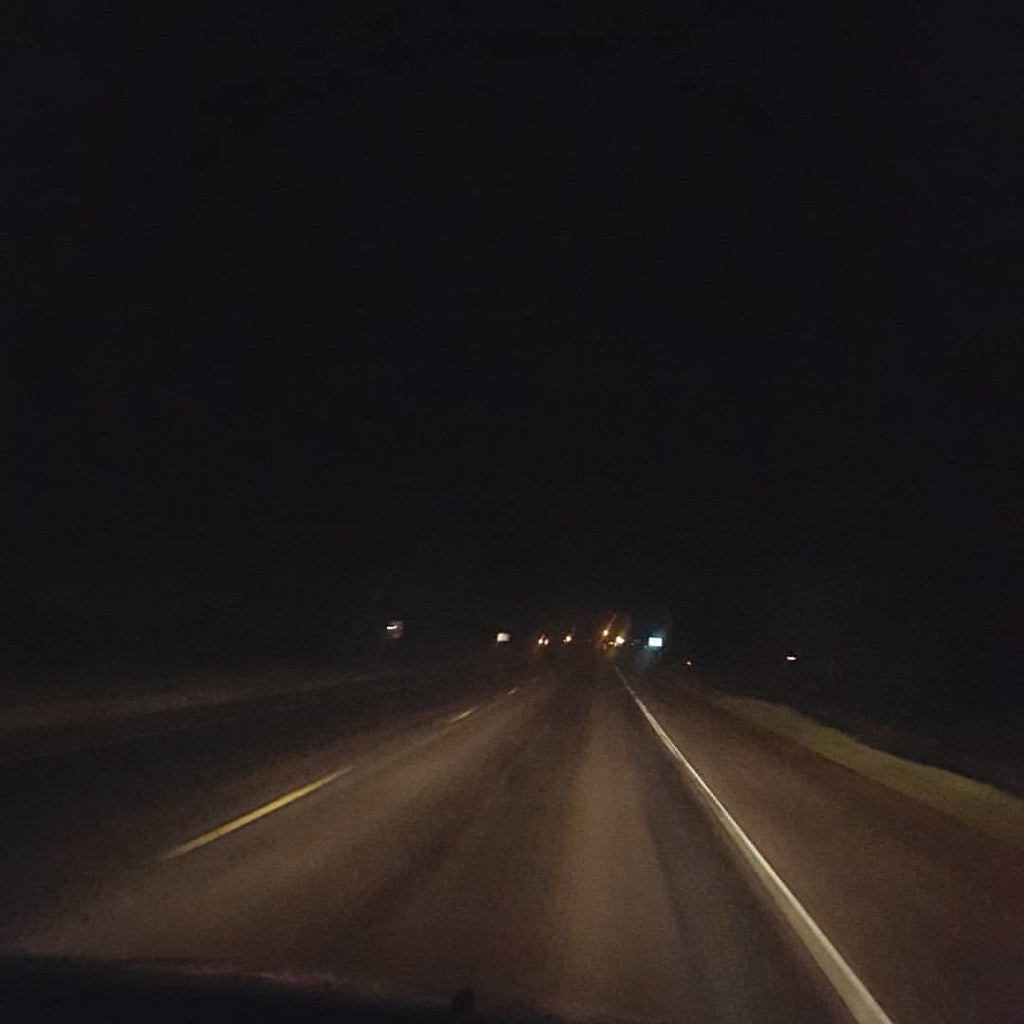This color photograph, taken at night from inside a vehicle, captures a dark, slightly out-of-focus view of a straight highway. The image is taken from the perspective of someone in the right-hand lane, likely a passenger, as indicated by the road's angle and the elongated, dark silhouette of what could be part of a car dashboard in the lower left corner. The photo is very dark, with little light illumination except for the stretch of roadway immediately in front, lit by headlights. The highway features a solid white line on the right and a dashed yellow line in the center. The upper two-thirds of the photo fade into darkness, with no visible streetlights or surrounding scenery. Distant lights, possibly from cars or reflective signs, punctuate the background, alongside what appears to be an illuminated rectangular road sign on the side of the highway. The image evokes a sense of isolation, with no other vehicles nearby and a clear, uninterrupted path ahead.